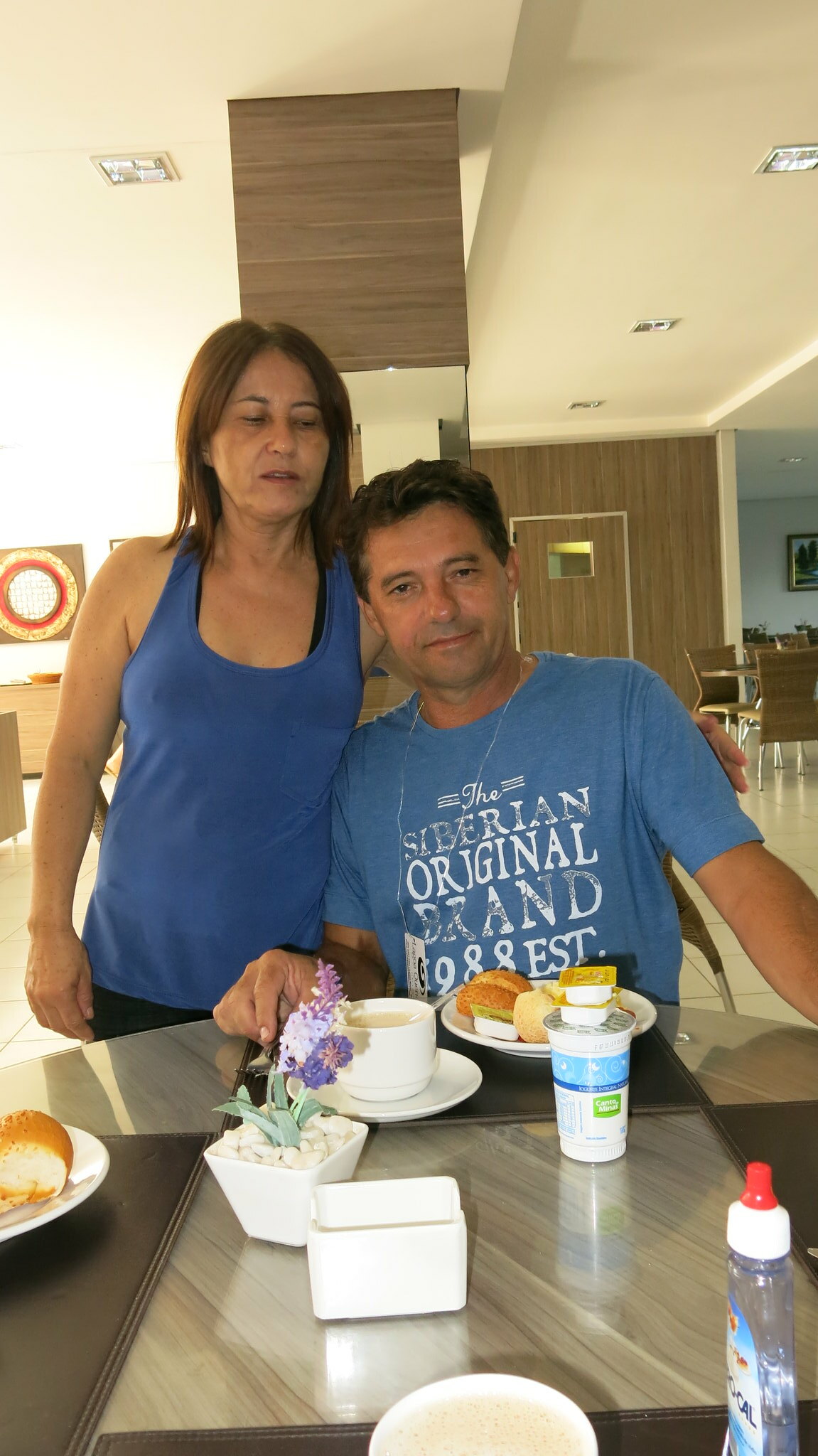This photograph captures a candid moment between a woman and a man in a homey kitchen setting. The woman, standing on the left, has short dark brown hair and is dressed in a blue v-neck shirt paired with black bottoms. Her eyes are either closed or looking downwards. The man, seated to the right, features short dark hair and is wearing a blue t-shirt with white text that reads "The Siberian Original Brand 1988 Established." He is accessorized with a silver necklace and is gazing into the camera. The table he is sitting at is round and gray, adorned with numerous breakfast items. Directly in front of him, there is a plate with bread and butter, a large cup of coffee, and a saucer. He holds a silver fork in his hand. Additionally, the table setting includes a little white vase with blue, purple, and lavender flowers, a white cup with a blue stripe holding two packets, possibly butter, another plate with bread and butter, a round dish with an indiscernible item, and a clear container with a white top and red spout. Behind the woman, there are some chairs arranged to her right, and a piece of art hangs on the left wall of the photo, featuring a mix of red and yellow circles with blue trim in the background.